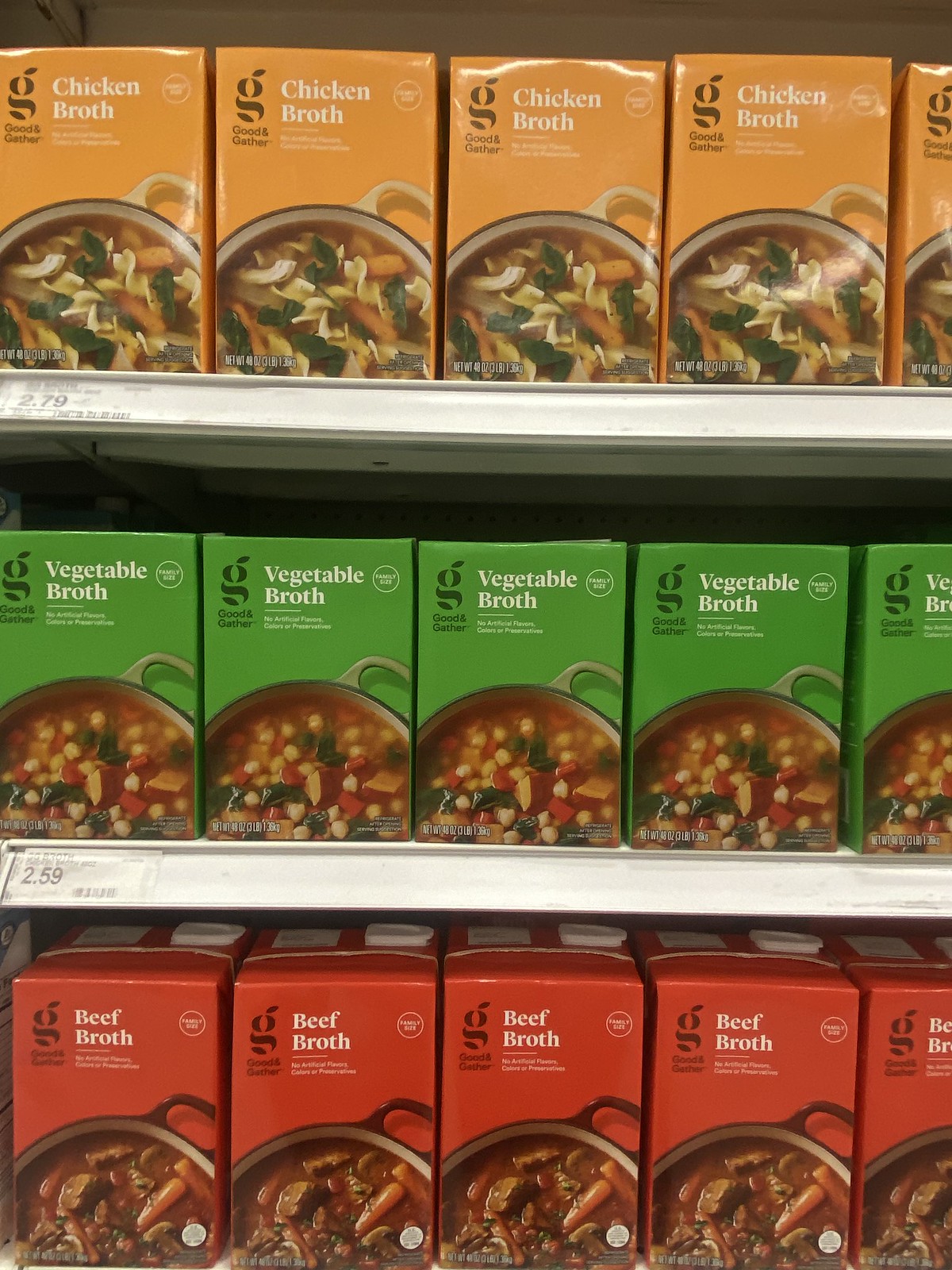This image captures a set of supermarket shelves meticulously stocked with a variety of broths. There are three distinct shelves, each dedicated to a specific type of broth. 

On the bottom shelf, red boxes of beef broth are prominently displayed, featuring an appetizing image of beef stew on the packaging. The middle shelf houses the vegetable broth, which is packaged in green boxes adorned with an image of what appears to be a hearty vegetable soup. The top shelf showcases orange boxes of chicken broth, each with an image that seems to depict a savory soup or pasta dish.

Each box, regardless of the type of broth, features the letter 'G' in the upper left-hand corner, accompanied by some text that is not easily readable.